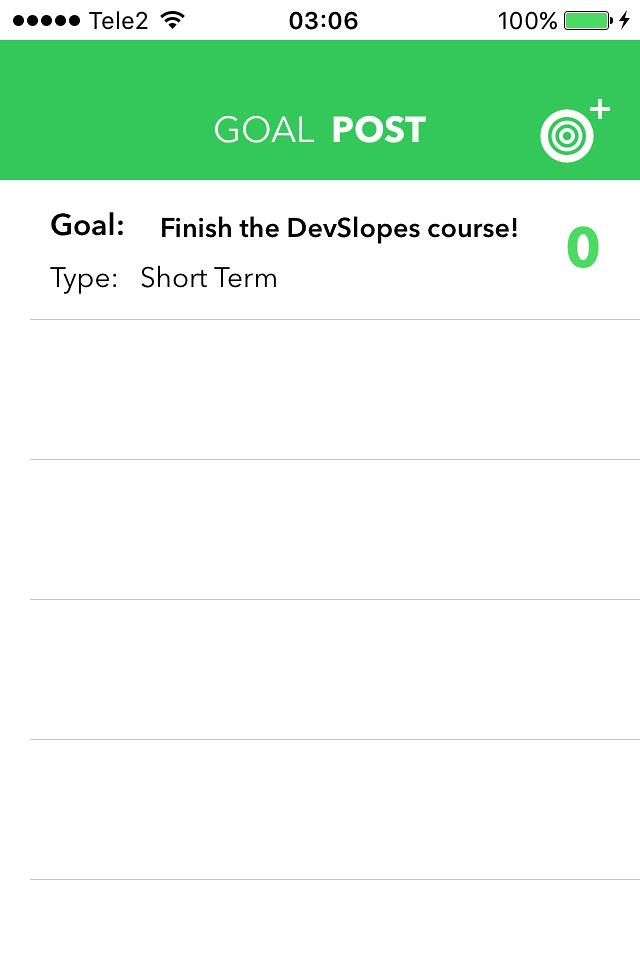The image captures a screenshot from a phone app. At the very top, the notification bar displays several icons for Wi-Fi, the text "Tally 2," the time "03:06," and the battery status showing 100% and charging. Below the notification bar, a light green banner features the bolded text "Goal Post," accompanied by a target icon with concentric circles and a plus sign. Further down, bold black letters state the goal: "Finish the DevSlopes course!" with "Type: Short Term" noted below in unbolded letters. A green number "0" is displayed to the right of this text. The rest of the screen contains five evenly spaced horizontal black lines, with no additional content.